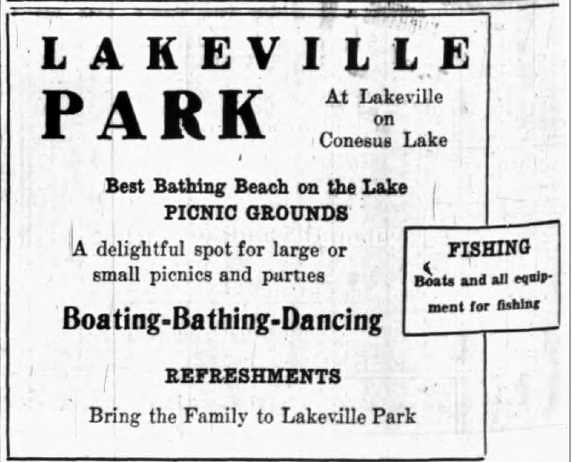This image showcases a vintage advertisement poster for Lakeville Park, located on Conesus Lake. The poster features black text on a slightly aged, whitish-gray background. Dominating the center of the poster, large black letters announce "Lakeville Park," followed by smaller text detailing the park's attractions: "At Lakeville on Conesus Lake," "Best Bathing Beach on the Lake," and "Picnic Grounds." Further, it highlights the park as "A Delightful Spot for Large or Small Picnics and Parties," and promotes activities like "Boating," "Bathing," and "Dancing," with "Refreshments" available. At the very bottom, it invites guests with "Bring the Family to Lakeville Park." A side box positioned towards the middle-right of the poster provides additional information about fishing, stating, "Fishing, Boats, and All Equipment for Fishing." The overall style of the advertisement suggests it is a nostalgic and weathered poster, evoking a sense of timeless family fun and outdoor recreation.